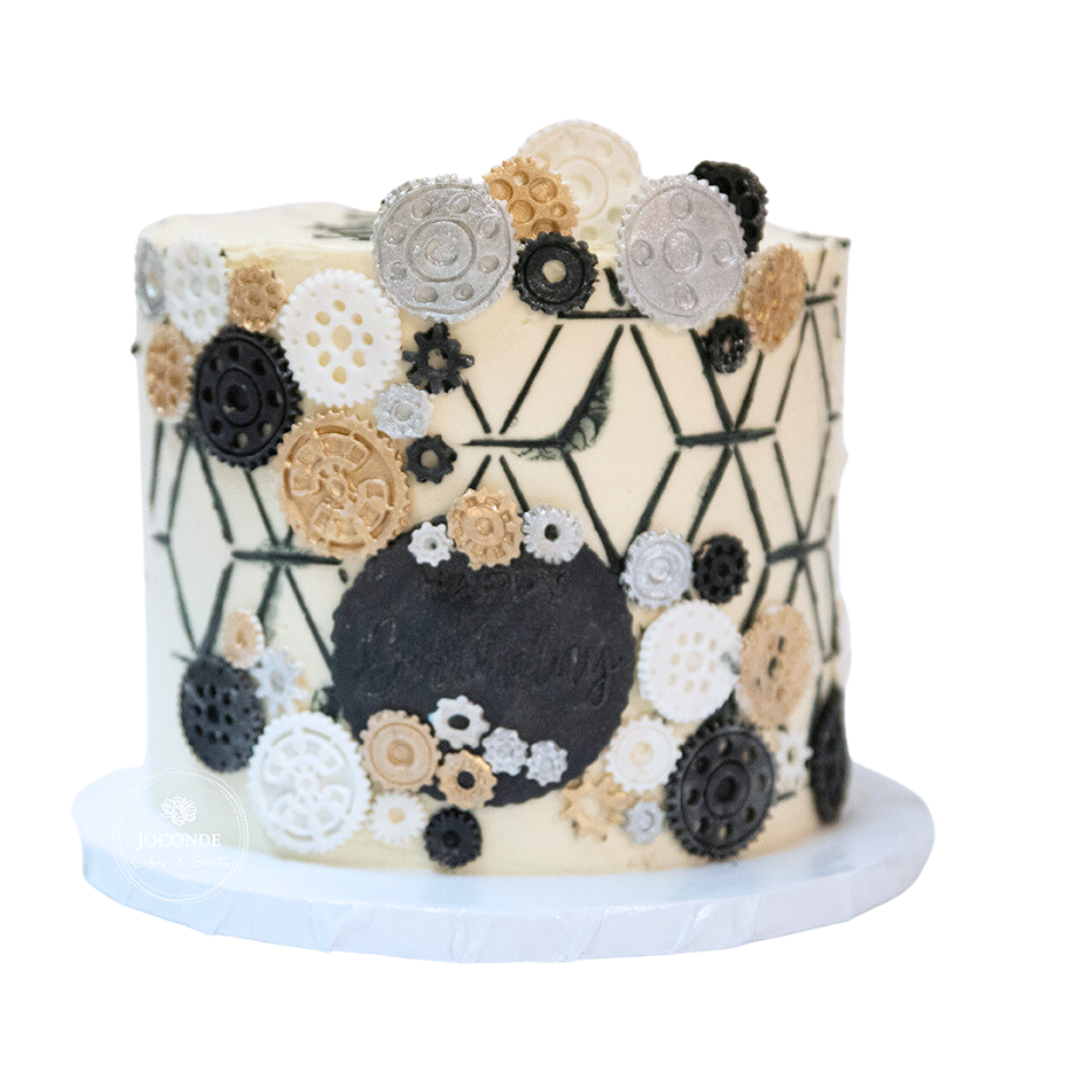The image depicts a medium-sized, cylindrical cake resting on a white circular base. The cake is covered in smooth, cream-colored fondant with a distinctive black diamond pattern adorning its sides. Scattered across the cake are various gear-shaped decorations in black, white, silver, and gold. These gears vary in size from tiny to extra-large and are randomly placed, adding an intricate touch to the design. The cake lacks any text or candles and is set against a plain white backdrop, emphasizing its detailed and elegant decorations.